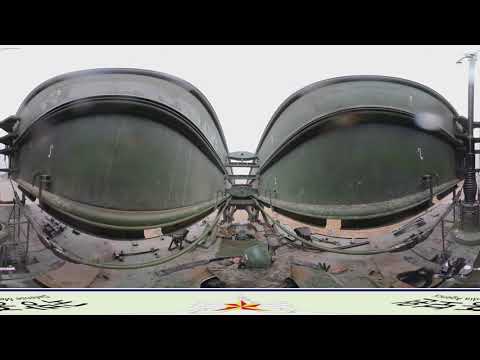This photo captures a highly distorted, possibly Photoshopped image of what appears to be military equipment or structure positioned outdoors. Two large, dome-shaped objects with darkish green, steel-like surfaces dominate the scene, possibly resembling cylindrical walls or large pipings. These structures curve and bend unnaturally, creating a warped 360-degree effect that emphasizes a central straight line flanked by these curved forms. The lower portions of these objects feature tan and rust hues, adding to the industrial or military look. In the foreground, there are black fixtures, possibly girders, running horizontally. The setting appears to be a parking lot with a few cars and a light post to the right, all beneath a bright, off-white sky. A glare is noticeable on the right side of the image, adding to the overall distortion. The bottom edge of the picture features unreadable lettering and a logo, further indicating some form of equipment or industrial complex.